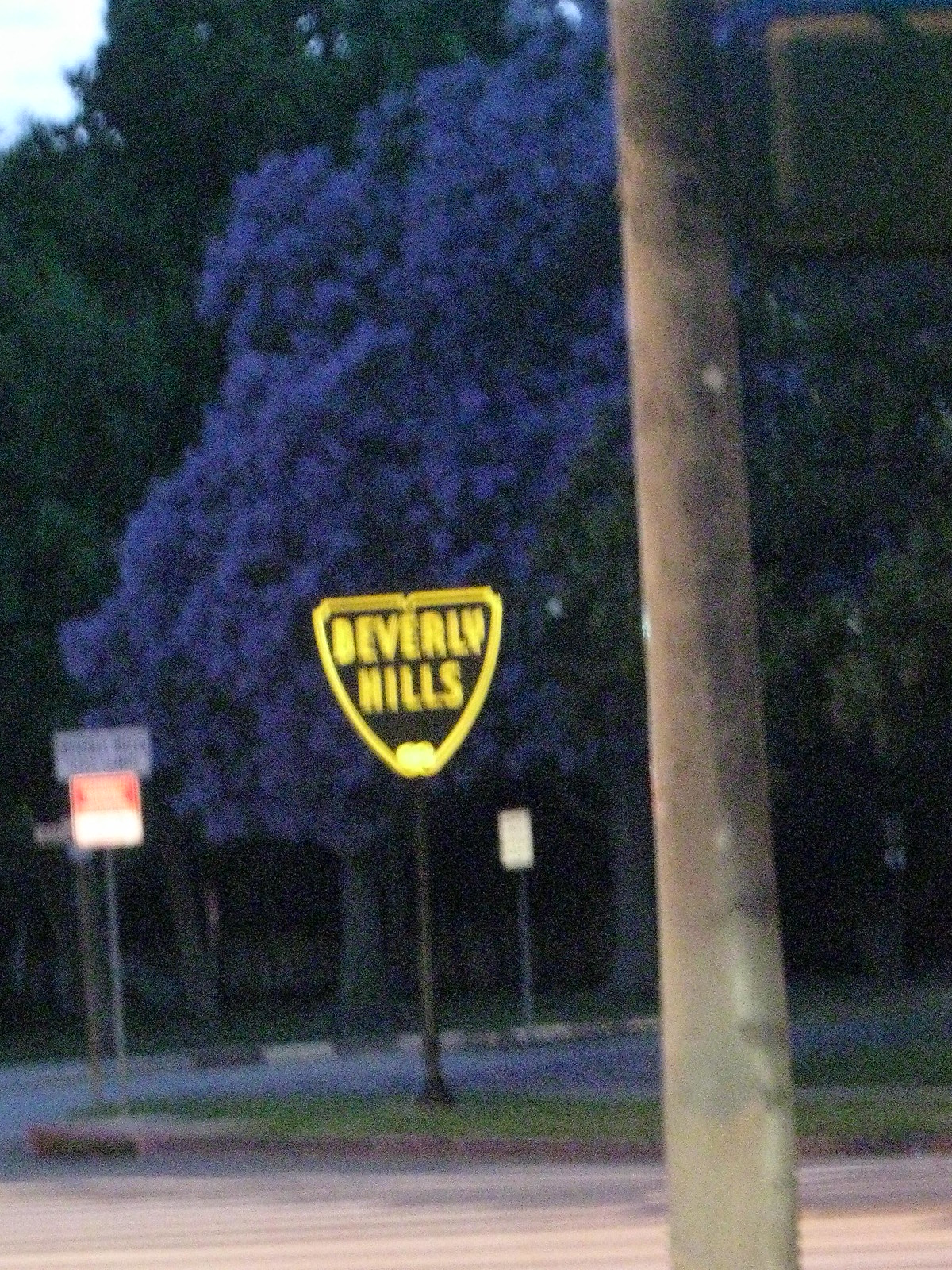The image depicts a bustling outdoor street scene with various signs and natural elements. Dominating the upper left-hand corner is a sliver of blue sky accented by a white cloud, suggesting it might still be sunny despite the overall darker tone of the image, making the time of day unclear. Prominently featured on the right side of the photo is a silver pole with a square pedestrian crossing signal affixed to it. Across the street, a black pole supports an upside-down yellow triangle sign, which reads "Beverly Hills" in yellow letters against a black background. Below this sign, a smaller street sign emerges. The scene showcases plentiful greenery, with trees filling up the upper half of the frame. Notably, one tree stands out with purple leaves amid the other green-leafed trees. Additionally, a brown tree trunk extends vertically along the right, contributing to the natural yet urban setting. Some street signs with red, white, and black colors add to the nuanced detail in this complex, layered photograph.